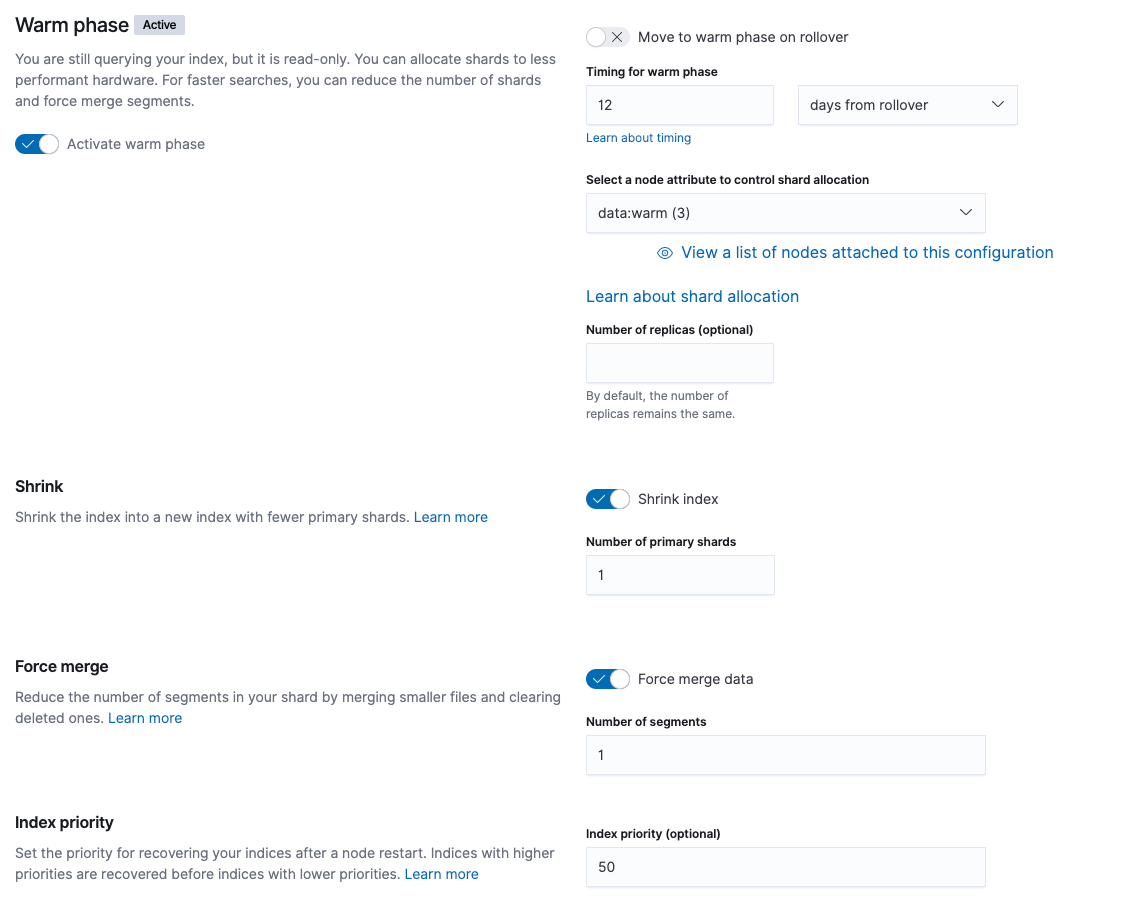Top Left: The phrase "Warm Face" is prominently displayed in a black, bold Arial font.

Top Right: A gray rectangle with a bluish tint houses the word "Active" centered in bold black font. Below this, in gray text, it states: "You are still querying your index, but it is read-only. You can allocate shards to less performant hardware. For faster searches, you can reduce the number of shards and merge segments."

Toggled Option: There is a toggle switch that is in the 'on' position, indicated by a white circle on the right side of a dark blue oval and a white check mark on the left. Adjacent to this, in gray, it reads "Active Warm Face."

Center of the Page, Towards the Bottom: 
1. A section titled "Shrink" appears in bold black lettering. Beneath this title, in light gray font, it says: "Shrink the index into a new index with fewer primary shards. Learn more." The "Learn more" text is blue, indicating a clickable URL.
   
2. Another heading, "Force Merge," is also in black bold font. Below it, in light gray, it explains: "Reduce the number of segments in your shard by merging smaller files and clearing deleted ones. Learn more." Once again, "Learn more" is blue and clickable.

Bottom Section:
3. A header titled "Index Priority" appears in black bold font. Its description, in gray text, reads: "Set the priority for recovering your indices after a node restart. Indices with higher priorities are recovered before indices with lower priorities. Learn more." The "Learn more" text here is also blue and clickable.

This detailed caption encapsulates the layout and contents of the image, translating the visual and textual elements into a comprehensive description.